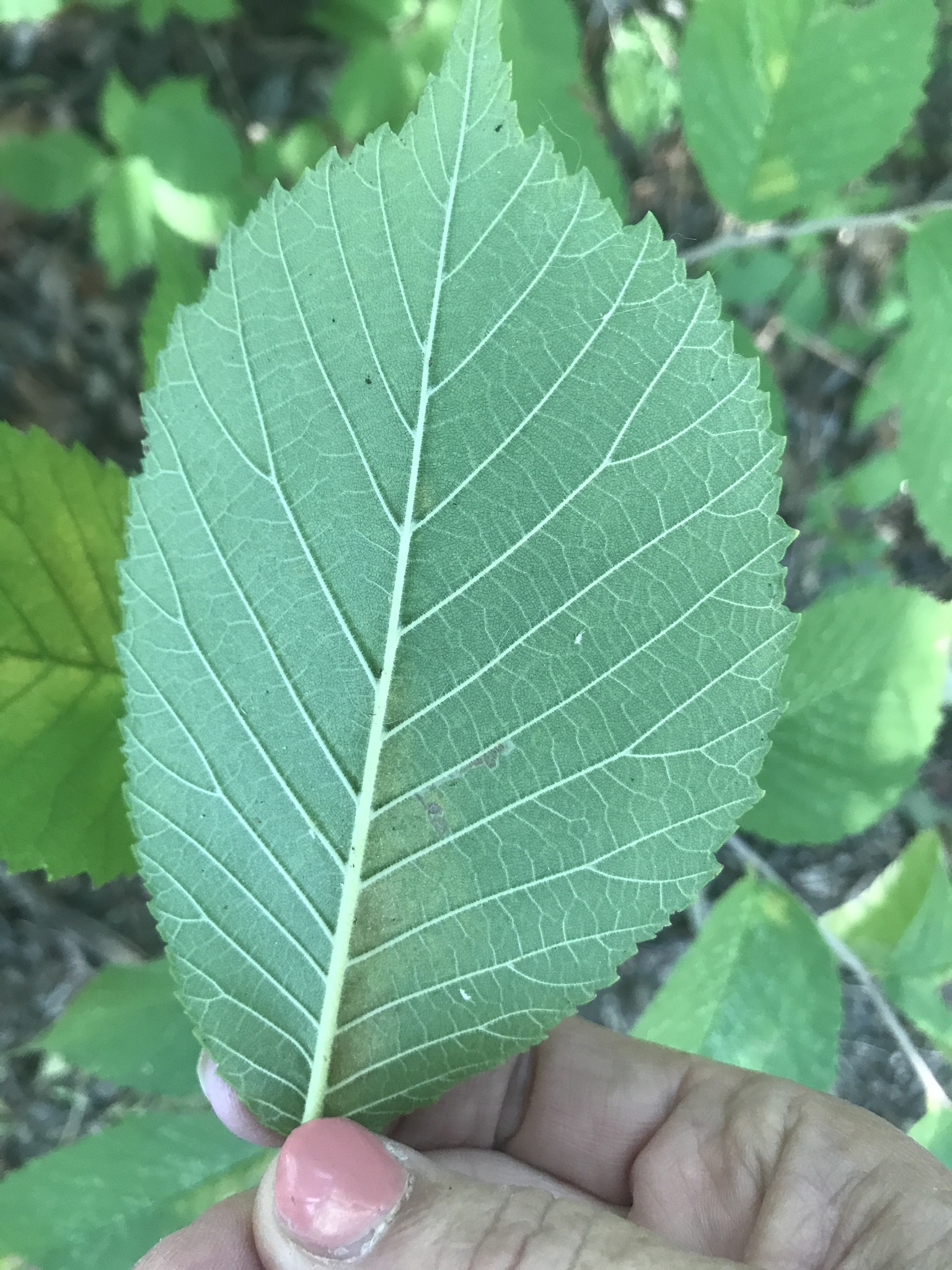In this detailed photograph, prominently captured in portrait mode, a freshly plucked, oval-shaped green leaf is delicately held by a darker-skinned person with well-worked hands adorned with pink nail polish. The forefinger and thumb, slightly wrinkled, firmly grip the light green stem at the base of the leaf. The photo emphasizes the intricate details of the leaf's back, showcasing the network of veins radiating outward, which highlight its lush, green texture. The blurred background features an assortment of leaves and stems in various shades of green and yellow, with a cluster of small black dots visible in the top left corner, enhancing the focus on the single leaf in the foreground.